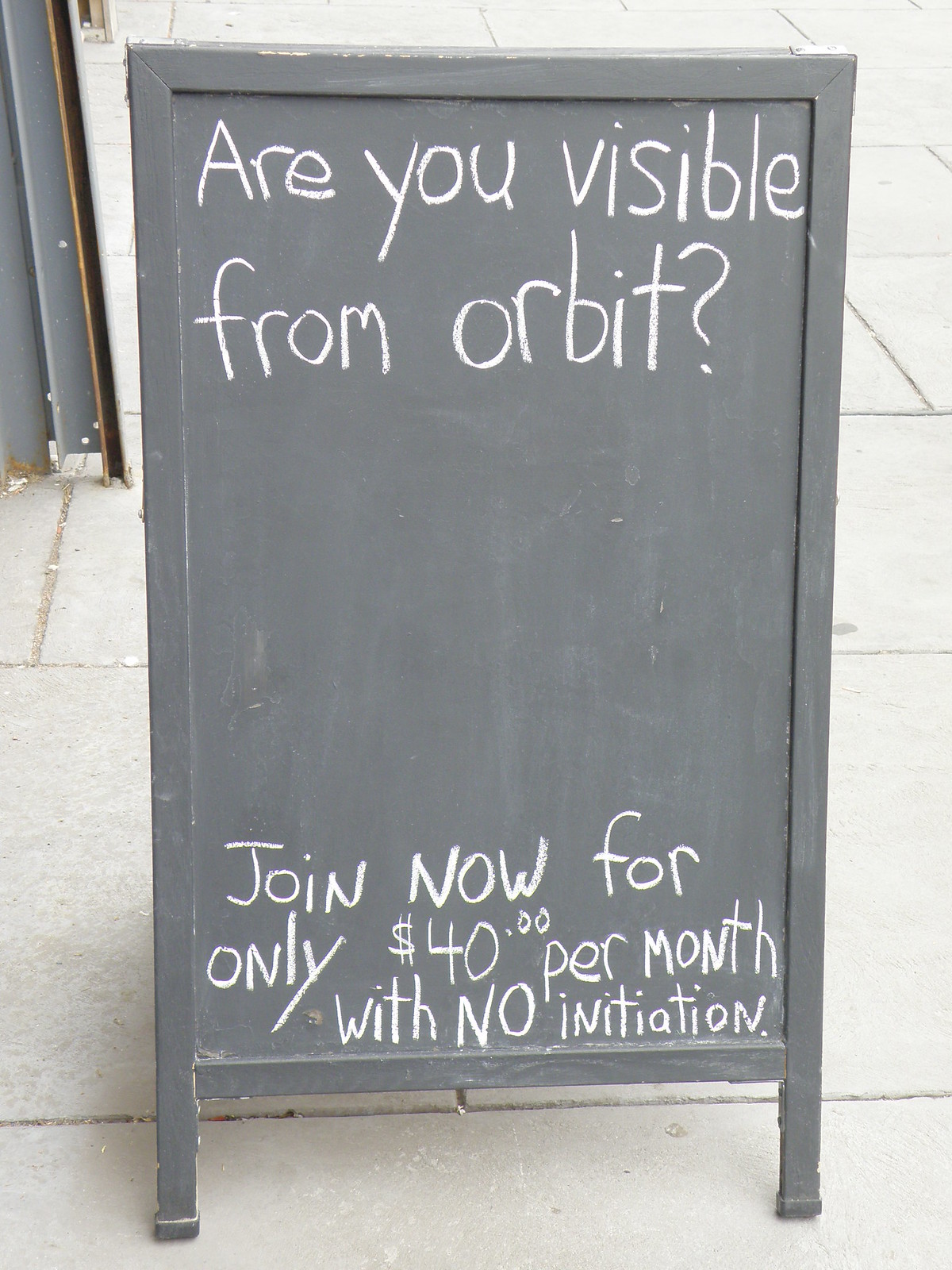The photograph is a bright, daytime outdoor shot of a gray wooden sandwich board, styled like a chalkboard, set up on a white concrete sidewalk in front of an unknown establishment. Written in white chalk, the sign poses the question, "Are you visible from orbit?" followed by the promotional offer, "Join now for only $40 per month with no initiation." The lettering is handmade, featuring a significant question mark. No people are present in the photograph, and it appears both the sign and the photo itself are relatively new. To the left of the sign, a metal door frame with fasteners, possibly a security shutter mechanism, is visible. There are no specific identifiers such as a date, location, or the name of the business advertised. The image is approximately 3x5 inches in size, offering a clear and detailed view of the scene.